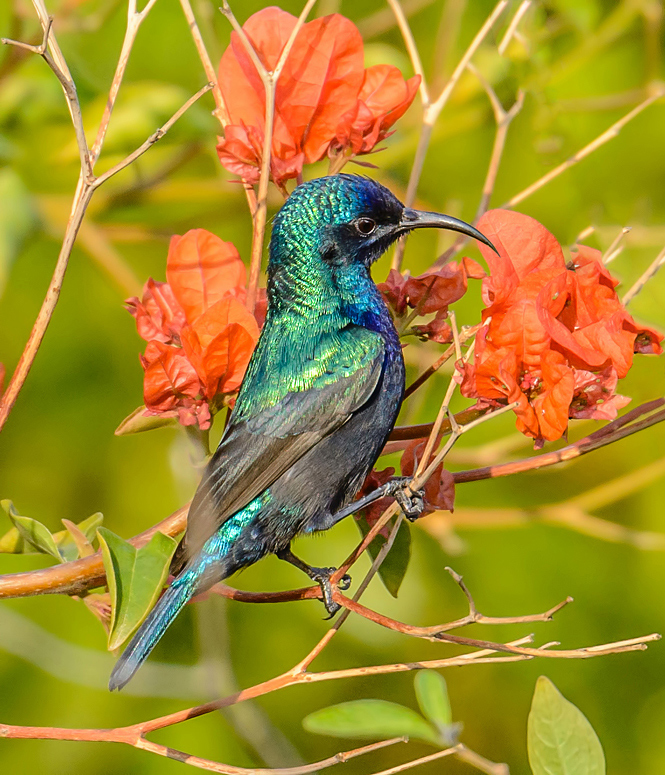In this detailed nature shot, we find a stunning, iridescent bird perched on thin, light brown branches, accentuated by vivid orange and red flowers. The bird, centered within the frame, showcases a mesmerizing blend of shiny blue, teal, and light green feathers. Its front, chest, and lower back are a deeper royal blue, while the tips of its wings exhibit a striking black hue. The bird's black feet are positioned with one slightly forward on the branch, and it features a distinct curved black beak. The setting is an outdoor scene with a blurred green background, giving hints of leaves and branches, emphasizing its natural habitat. The flowers are positioned thoughtfully around the bird, with one to the left, one directly above, and one to the right, enhancing the composition of this tranquil yet vibrant image.